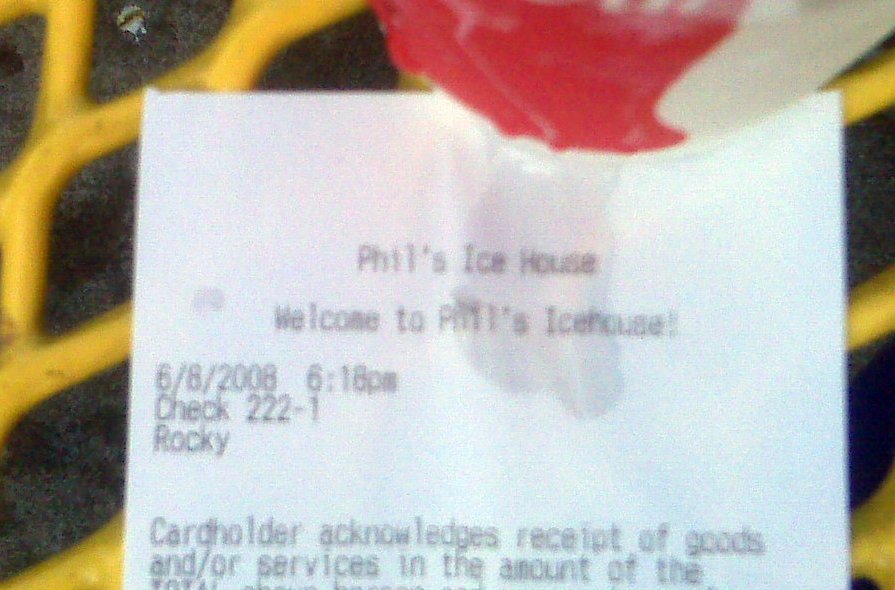The image is a close-up photograph of the upper portion of a receipt from Phil's Ice House, dated June 8th, 2008, at 6:18 PM. The receipt, which appears to be slightly stained by a liquid at the top, reads "Welcome to Phil's Ice House." The check number is 222-1, and it lists the name "Rocky," potentially hinting at an ice cream flavor such as Rocky Road. The partial legal statement at the bottom starts with "Cardholder acknowledges receipt of goods or services in the amount of..." and is cut off. The receipt is set against a background featuring a yellow surface with black diamond shapes, resembling a table with perforations typical of park furniture. A red and white spherical object and a watermark are also visible, along with what appears to be a finger with red nail polish holding the receipt.